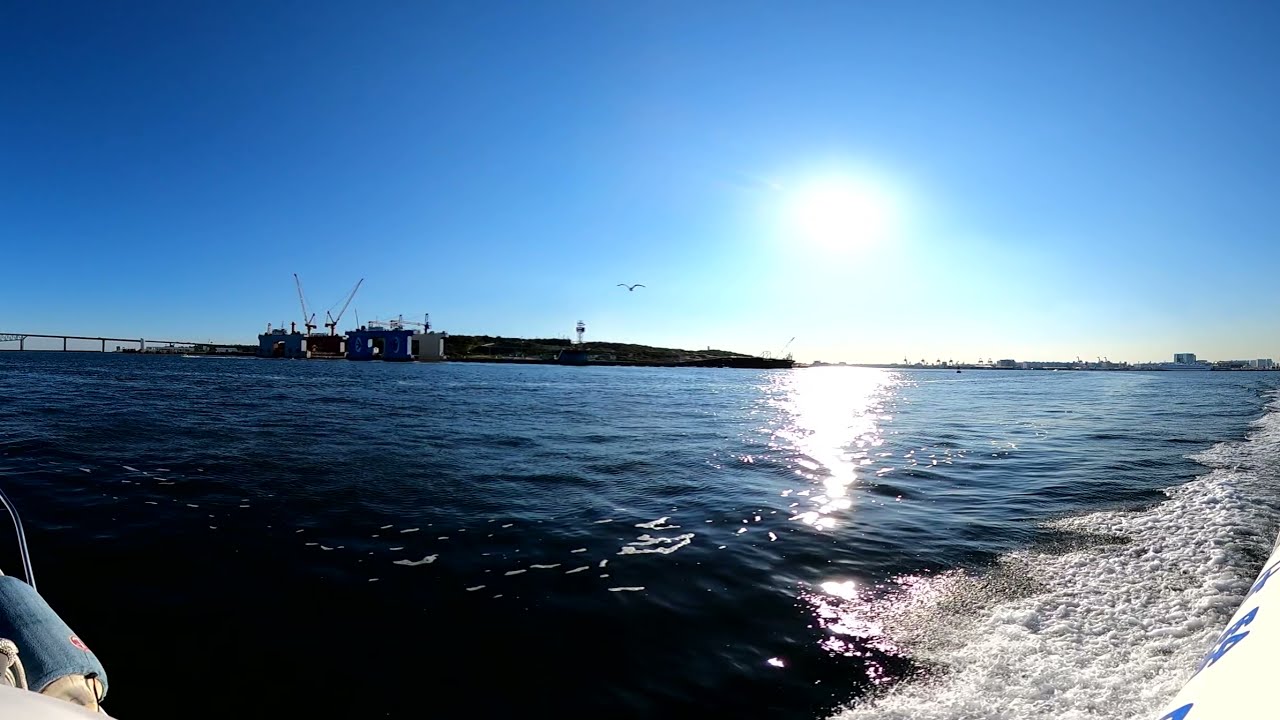The image captures a stunning vista of a large, clear blue body of water, most likely the ocean, taken from a boat. The sun shines brightly, casting a glowing white streak of light across the water and creating sparkling reflections. The presence of foamy waves and bubbles along the bottom right of the image signifies the boat's movement. The sky is an ombre gradient of blue, clear and free of clouds, enhancing the daytime setting. On the left side of the image, a bridge stretches across the horizon, while to the right, buildings in the distance become visible, suggesting a distant city. In the middle ground, there's a land mass with manufacturing or dock machinery, possibly a jetty or port, adding to the industrial backdrop. Additionally, a single bird is captured flying in the sky.